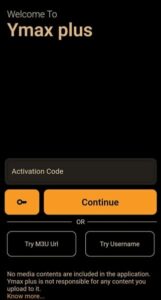A low-resolution, portrait-oriented screenshot from a mobile smartphone app displays a solid black background. In the top left corner, light grey text reads "Welcome to," followed by larger dark yellow text that says "Wimax Plus." Below, there's a large unused black area. About halfway down the screenshot, a brownish-grey box with a black outline contains small white text stating "Activation Code."

Beneath this, two dark yellow boxes are positioned side by side. The smaller, nearly square box on the left features a black key symbol. The larger, rectangular box on the right spans the rest of the screen width, bearing the word "Continue" in black text at its center.

A thin white dividing line follows these boxes, with the word "or" in white text centered on the line. Below this, after a short black gap, are two equally sized white-bordered rectangles with black interiors matching the background color. The first rectangle contains white text that says "Try M3U URL," while the second rectangle to the right reads "Try Username."

After another short gap, low-resolution white text states, "No media contents are included in the application. Wimax Plus is not responsible for any content you upload to it." Additionally, in orange text, the disclaimer ends with "No more..."